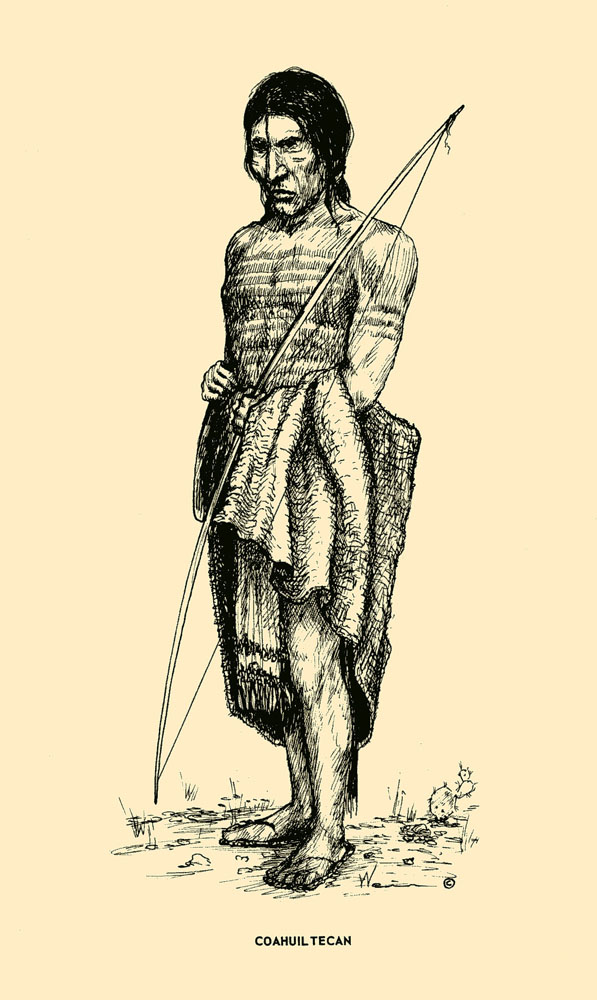This detailed sketch depicts a Native American man standing against a light pink, almost peach, background. The monochromatic illustration utilizes black and gray hues to create a vintage feel. The man has long, dark hair that flows down either side of his head and extends into a ponytail behind his back. His facial expression appears serious, potentially hinting at sadness. He is topless, revealing horizontal black stripes that stretch across his chest down to his stomach, suggesting tribal markings.

He holds a long bow, strung from the ground up over his head, slung over his left shoulder. His left hand, positioned in front of his chest, gently grasps a piece of drapery or cloth that folds over his forearm and hangs down, accentuating his slim build. Around his waist, he wears a gown-like garment, leaving his bare legs visible and highlighting his simple sandals, which feature woven straps between his toes.

The ground beneath him is textured with dirt, scattered grass, and a small cactus plant, contributing to the rustic atmosphere of the scene. Below the image, the words "Koahulil Tekan" are inscribed, though there are variations such as "Coahuilticon" and "Coahuiltecan" noted, emphasizing the cultural context of the portrayal.